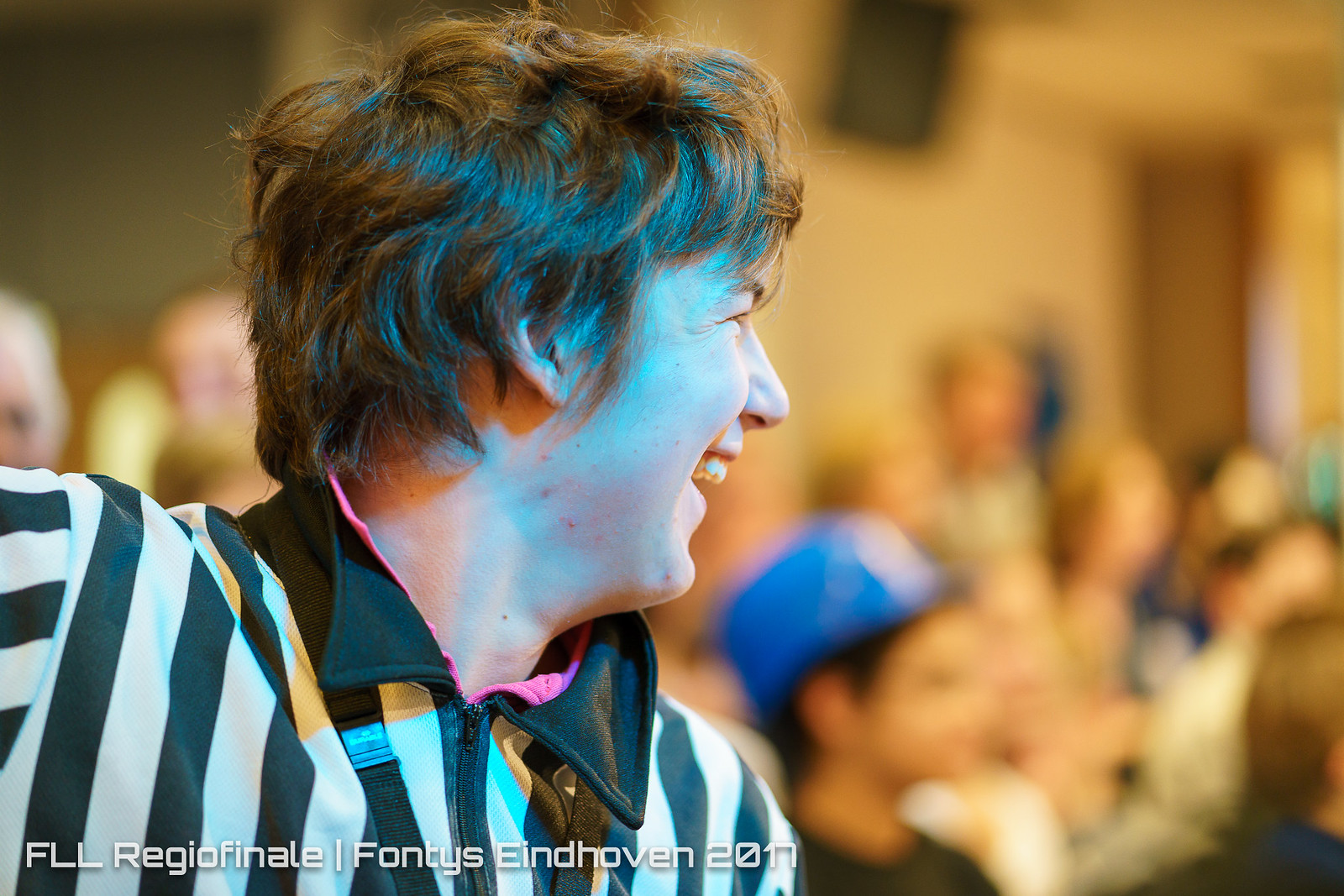The image captures a close-up of a person with unkempt long brown hair, turned to the right and laughing with visible teeth and squinting eyes. They are wearing a black and white vertically-striped shirt reminiscent of a referee's uniform. Positioned against a backdrop that suggests an indoor setting, possibly a gymnasium, the background is heavily blurred but populated with numerous people. Some background elements, such as a black ceiling speaker and a person wearing a baseball cap, can be discerned. The subjects in the background, though blurry, appear to be looking in the same direction as the central figure and seem to be smiling. On the bottom left of the image, white text reads: "FLL Regio Finale, Fontys, Eindhoven, 2017," adding context to the event's location and date.